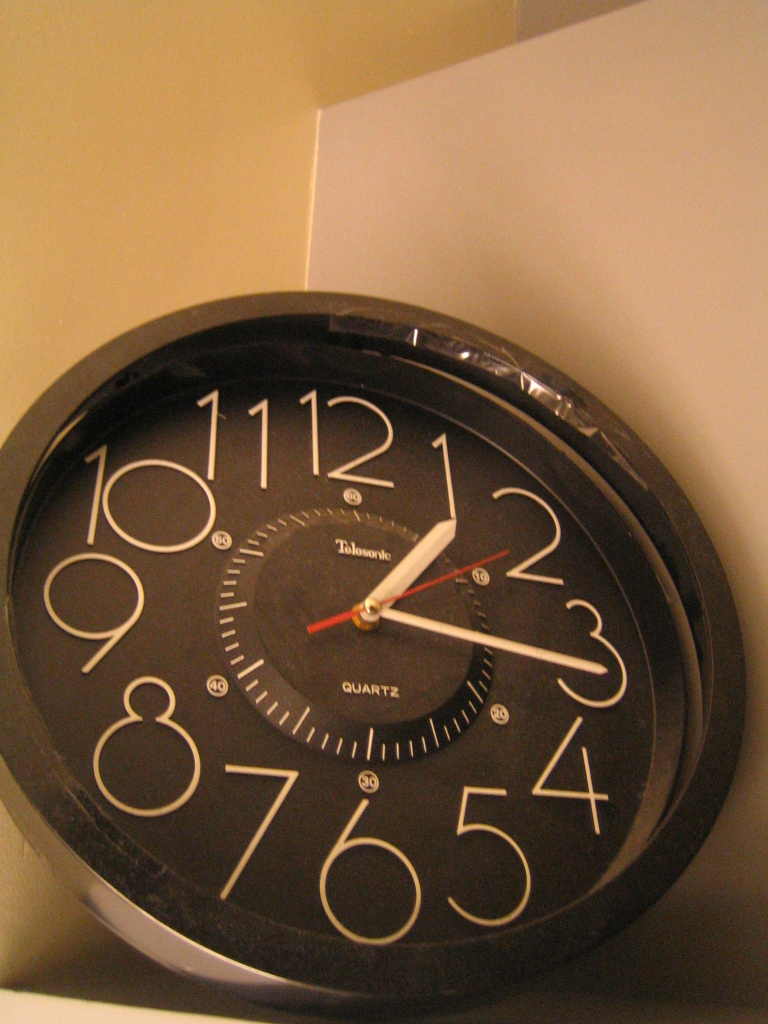The photograph features a close-up of a round, black clock positioned against a two-toned wall, with one section in beige and another in white. The clock, which resembles a portable tabletop model, has a silver metallic body with some clear tape on a portion of its case, indicating it is being held in place. It displays large white numbers and smaller minute markers on its black face, with the time stopped at 1:16 and 10 seconds. The hour and minute hands are white, while the second hand is red, pointing at the 2 o'clock position. The center of the clock's face contains additional minute markers, reminiscent of a safe dial. Below the number 12, there is an illegible brand name that appears to start with a "T," followed by the word "quartz."